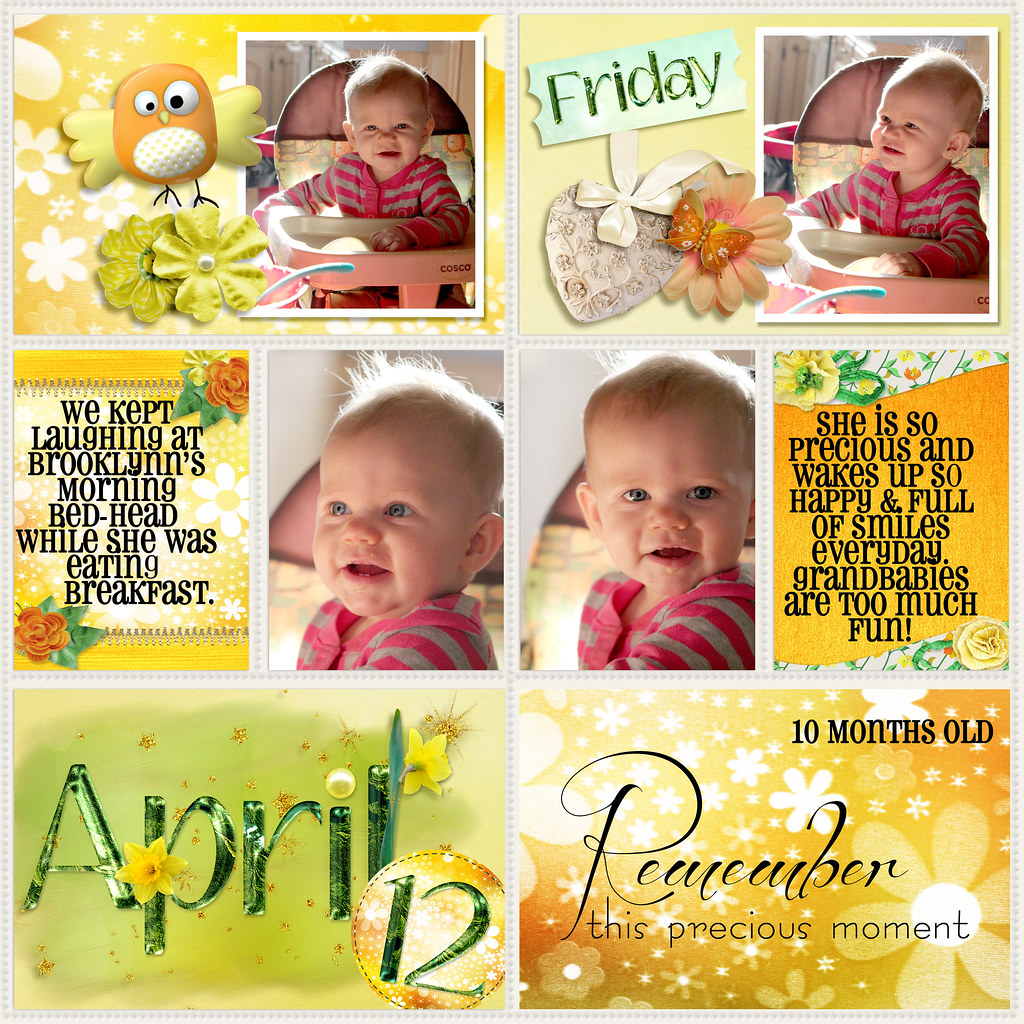The image is a detailed, six-section memory book montage. The top left section features a cartoon bird perched above two yellow flowers, set against a yellow background adorned with white flower outlines. A baby’s picture is framed within a white border beneath this colorful composition. Adjacent to it, the top middle section with the same yellow background has a banner in the top left corner labeled "Friday." Below this, a heart shape decorated with a flower and a butterfly encloses another baby photo. In the center left section, black text reads, "We kept laughing at Brooklyn's morning bedhead while she was eating breakfast." Four photographs of the same child in the same outfit, but different poses, are scattered throughout the montage, maturing the narrative of joyful moments with Brooklyn.